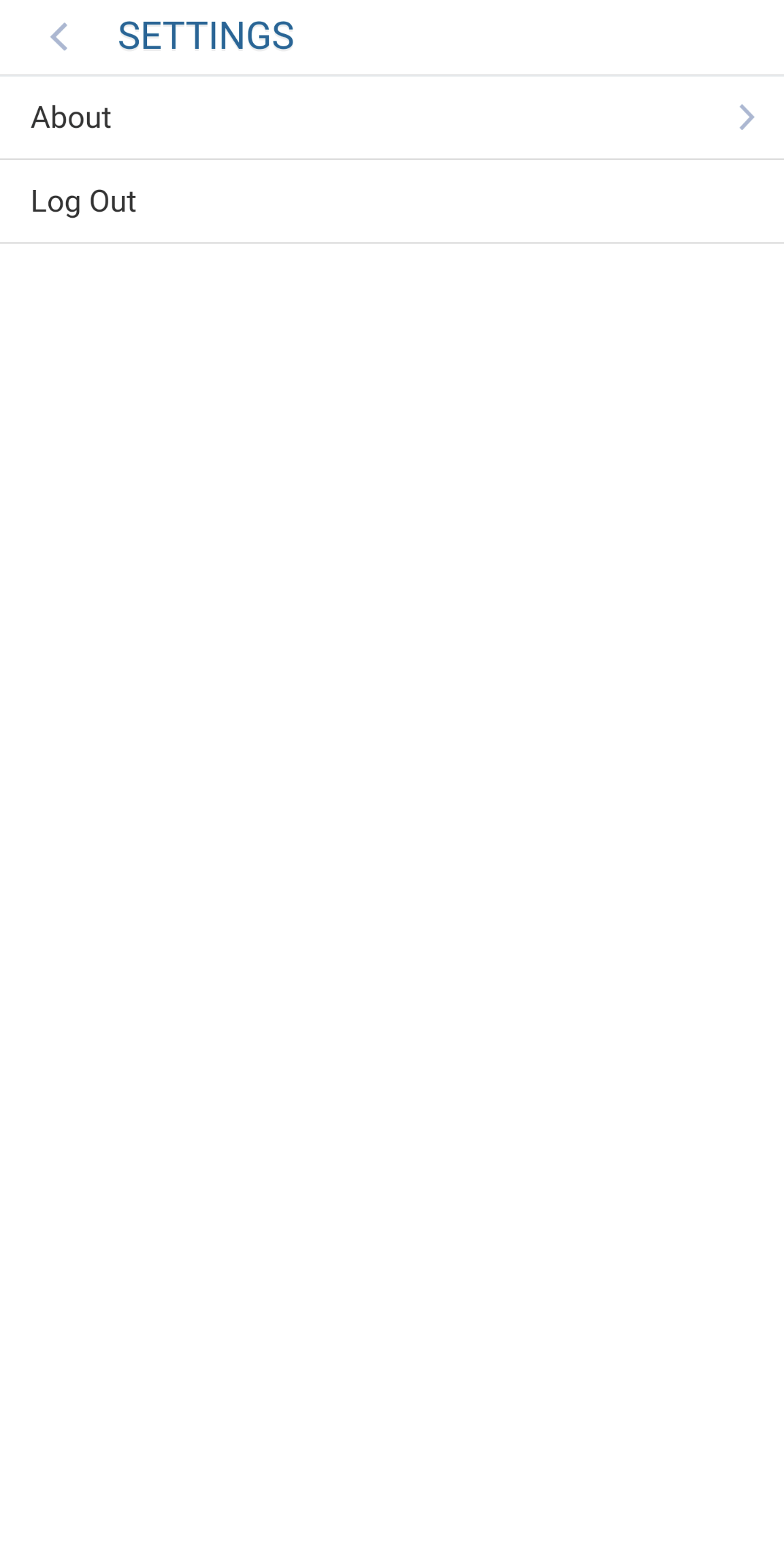In the image, the central focus is a user interface featuring a settings menu. On the right side of the menu, the word "Settings" is prominently displayed. Below this, a left-pointing arrow is visible, indicating navigation to a previous screen or menu. Directly beneath this symbol is the label "About," which is highlighted in black. To the right of "About," there's a right-pointing arrow suggesting that clicking it would expand further details or options. Below "About," the label "Log Out" is also highlighted in black. Notably, there is no additional contextual information provided to clarify whether this settings menu belongs to a phone, a computer, or another device, making it ambiguous. Thus, the exact origin or specific application of these settings remains unclear, adding an element of mystery to the overall scene.